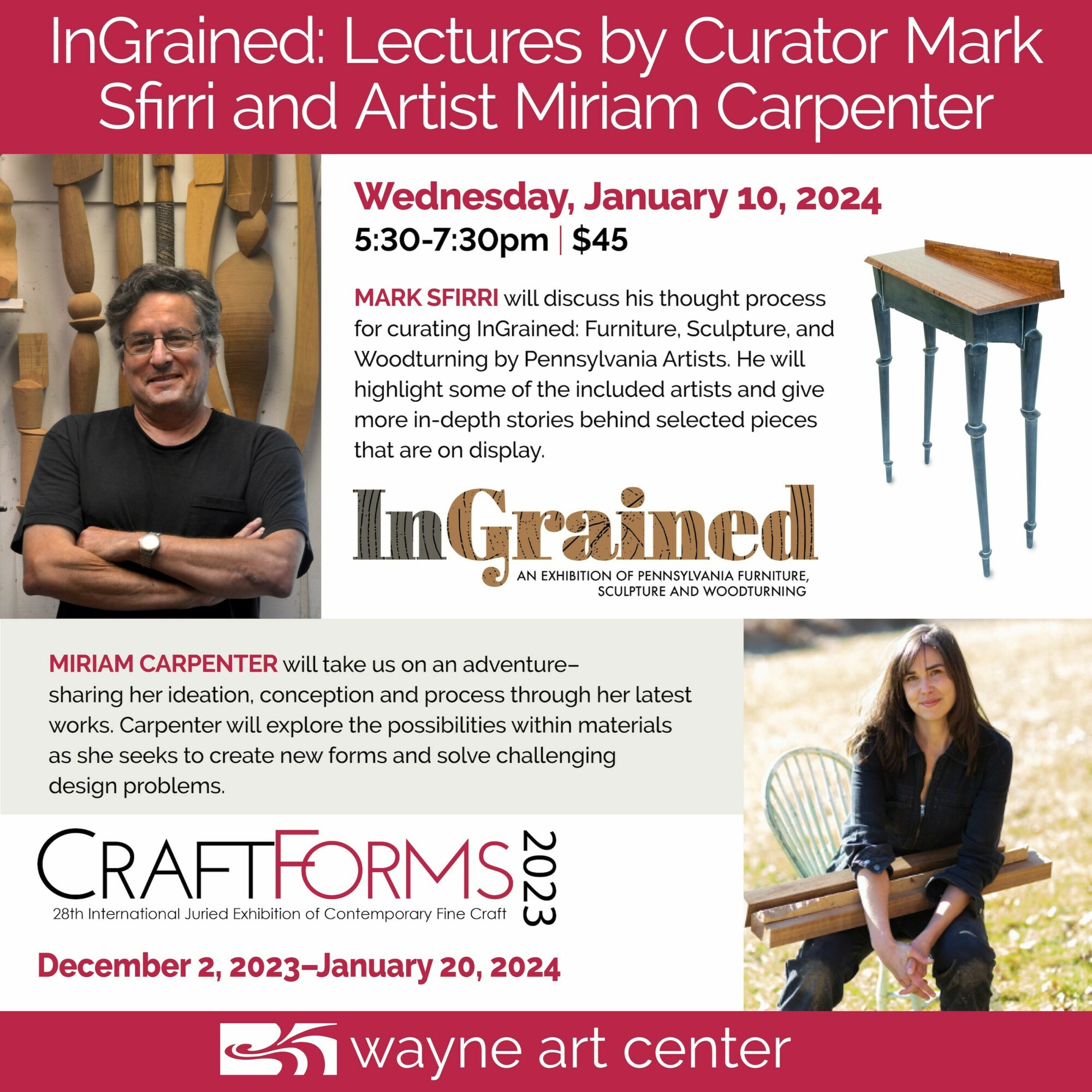This poster advertises "Ingrained Lectures" featuring Curator Mark Sfiri and Artist Miriam Carpenter, presented by Craft Forms 2023 at the Wayne Art Center from December 2nd, 2023, to January 20th, 2024. At the top, within a red box with white text, it reads "Ingrained: Lectures by Curator Mark Sfiri and Artist Miriam Carpenter." Below this, on the left, there is a photograph of Mark Sfiri, smiling with folded arms, wearing a black t-shirt and glasses. To the right of his image, details of his lecture are provided: "Wednesday, January 10th, 2024, 5:30 to 7:30 p.m., $45." Sfiri will discuss his thought process for curating ingrained furniture, sculpture, and woodturning by Pennsylvania artists, highlighting some artists and delving into the stories behind selected pieces on display. Below that, in a larger font, the word "Ingrained" is displayed prominently. Below this, in a light gray box, text describes Miriam Carpenter's lecture: she will take the audience on an adventure through her ideation, conception, and creative process, exploring new possibilities within materials and solving challenging design problems. Carpenter's photograph is situated at the lower right; she is seated on a chair, smiling with her hands clasped, wearing a black outfit. At the very bottom of the poster, in another red box, it reads "Wayne Art Center."